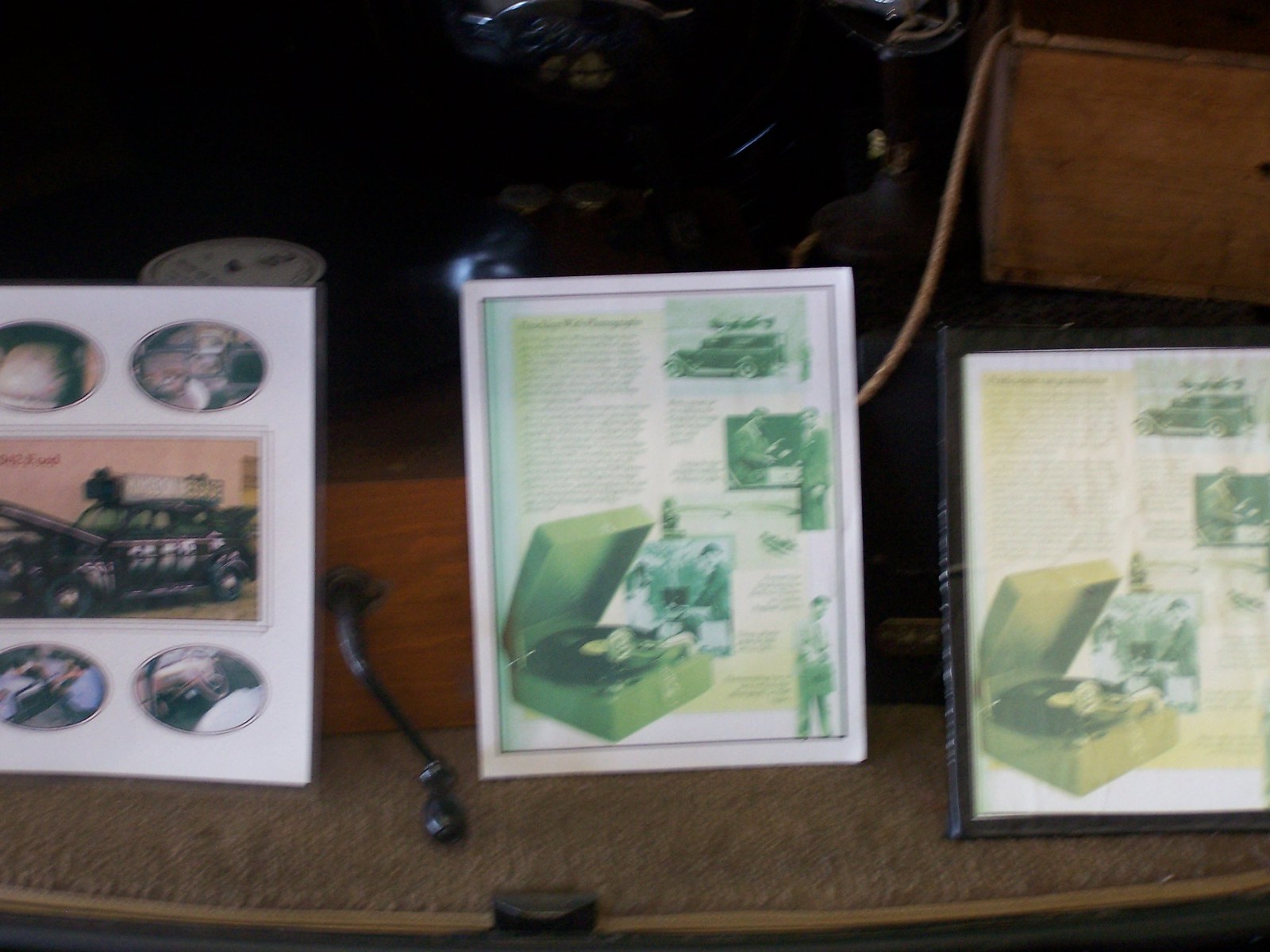This photograph depicts a museum or function display featuring vintage technology, specifically focusing on a record player. Centered in the background is a brown box with a crank and metal lock handle on the front, partially shadowed but revealing a white-labeled record within. A brown cord extends from the box’s right side. The display is arranged on light brown tan carpeting or circular cloth lining. In front of the record player, three horizontally aligned papers are propped up. Two papers appear identical and detail diagrams of the phonograph, while the third paper on the left showcases multiple blurry images of an old car, including exterior shots and the steering wheel. The papers exhibit slight color variations, with green and yellow tinges. Additional indistinct items and images lean against wooden boxes to the right, further enriching the exhibition setup.